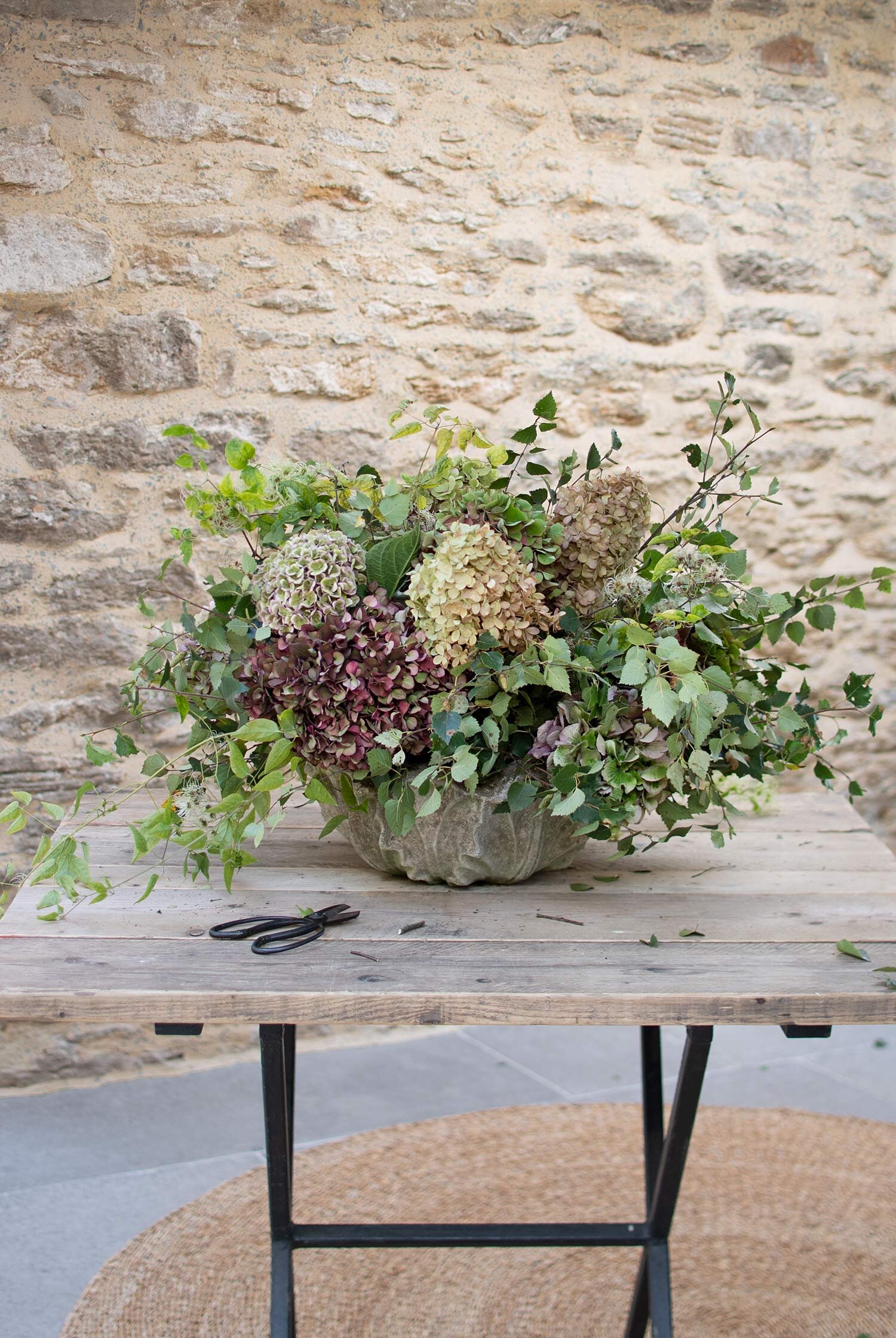In this photograph, a light wooden table with black legs, featuring two black hooks on its underside, is prominently displayed. The table supports a pot that looks like porcelain and stone designed to mimic a cabbage, containing a vibrant floral arrangement. The bouquet consists of an array of colorful carnations in shades of pink, red, yellow, white, and beige, interspersed with lush green leaves that spill out over the pot. Additionally, there are muted purple, yellow, and red flowers, with most of the arrangement dominated by greenery. Beside the floral arrangement lies a small pair of black cutting scissors, giving the scene a touch of practicality. The background features a beige and gray stone wall, while the floor is gray concrete, possibly marble. Adding a cozy element, a circular light brown and beige mat, potentially made from rope, is placed on the floor beneath the table.